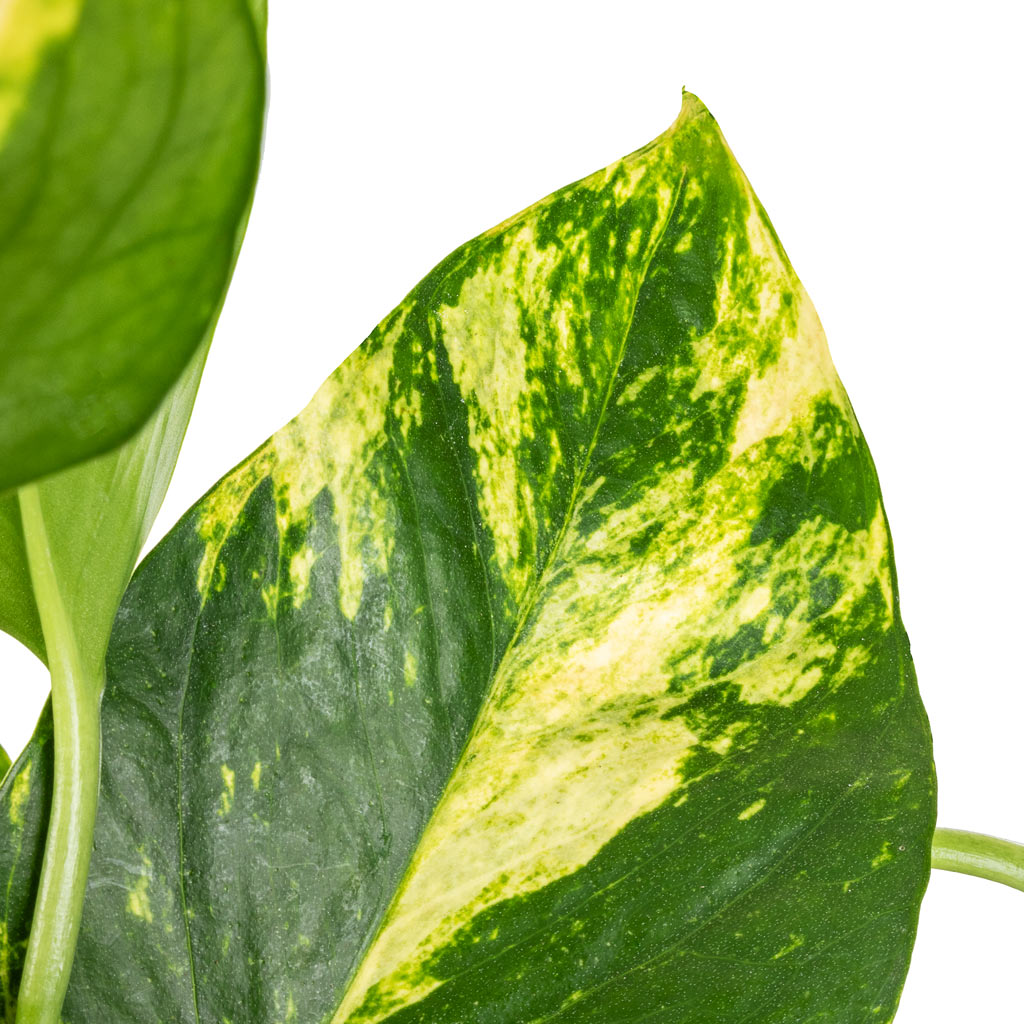A detailed close-up photograph features multiple overlapping leaves against a plain, pristine white background. The prominent central leaf is a dark green philodendron variegated with splatches of light green to yellow, showcasing a distinct pointy curve and a small tip at its rounded end. Veins run through this main leaf, with a central vein branching out symmetrically to the left and right, creating an intricate vascular pattern. To the left of this central leaf extends a visible stem, supporting areas of solid green and contrasting variegation. In the upper left corner, part of a third leaf emerges, displaying a similar variegated pattern. On the right side of the image, a solitary green stem is present, contributing to the overall composition, evoking a sense of natural beauty and botanical intricacy.